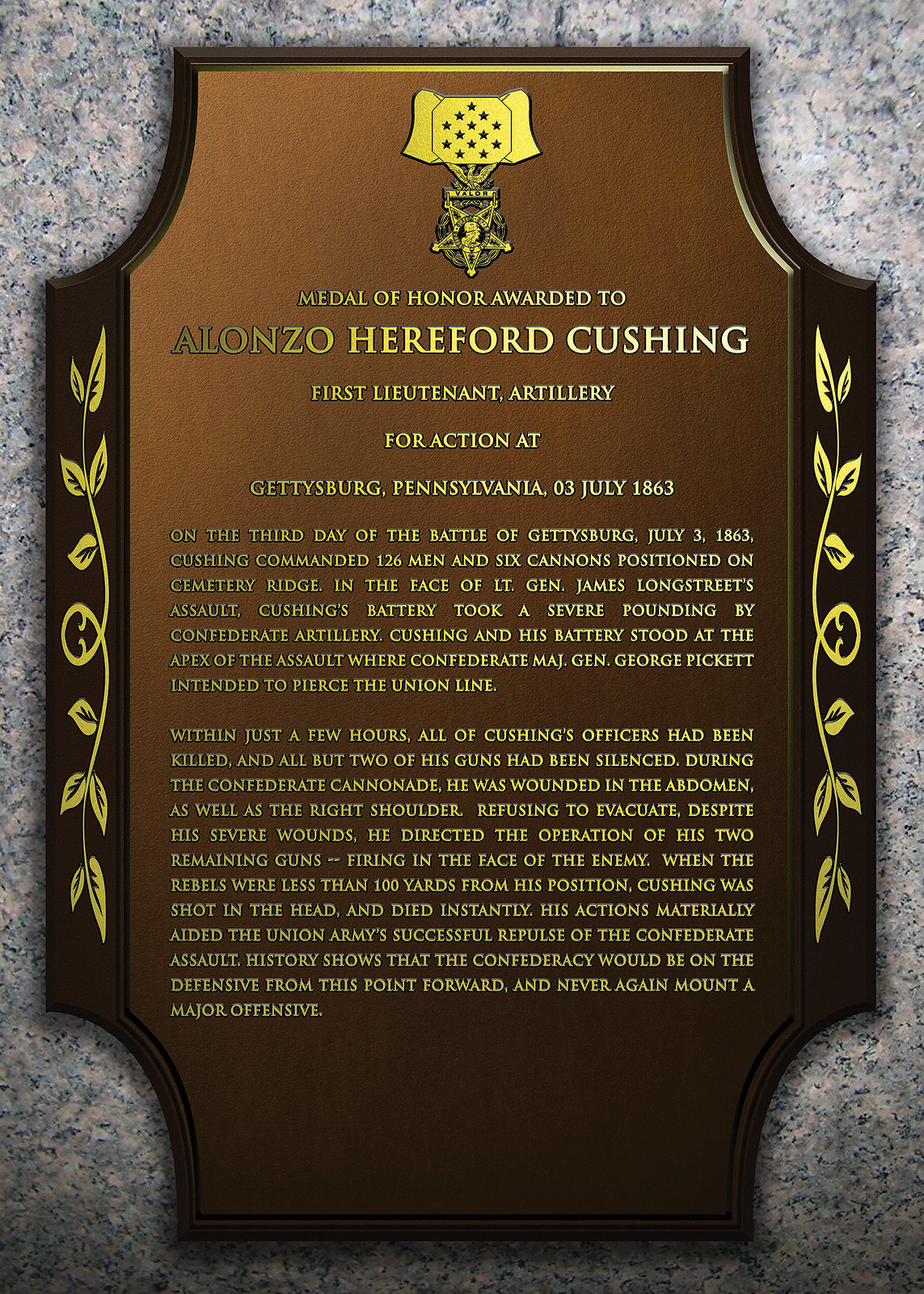The image portrays a detailed plaque honoring 1st Lieutenant Alonzo Hereford Cushing for his heroic actions during the Battle of Gettysburg on July 3, 1863. Mounted against a marble wall, the plaque features a brown base with darker brown sides, adorned with an intricate gold vine motif on each side. At the top, a distinguished Medal of Valor emblem is displayed. The engraved gold lettering reads:

"Medal of Honor awarded to Alonzo Hereford Cushing, 1st Lieutenant Artillery for Action at Gettysburg, Pennsylvania, 03 July 1863."

The plaque includes an in-depth narrative of Cushing’s valor during the battle. On the third day of the Battle of Gettysburg, Cushing commanded 126 men and six cannons at Cemetery Ridge. Despite severe losses and multiple injuries, he refused to evacuate and continued directing his remaining artillery until he was fatally shot, which significantly contributed to the Union Army’s successful defense. This pivotal moment marked the beginning of the Confederacy’s strategic decline. The polished juxtaposition of modern craftsmanship with historic valor beautifully encapsulates Cushing's enduring legacy.